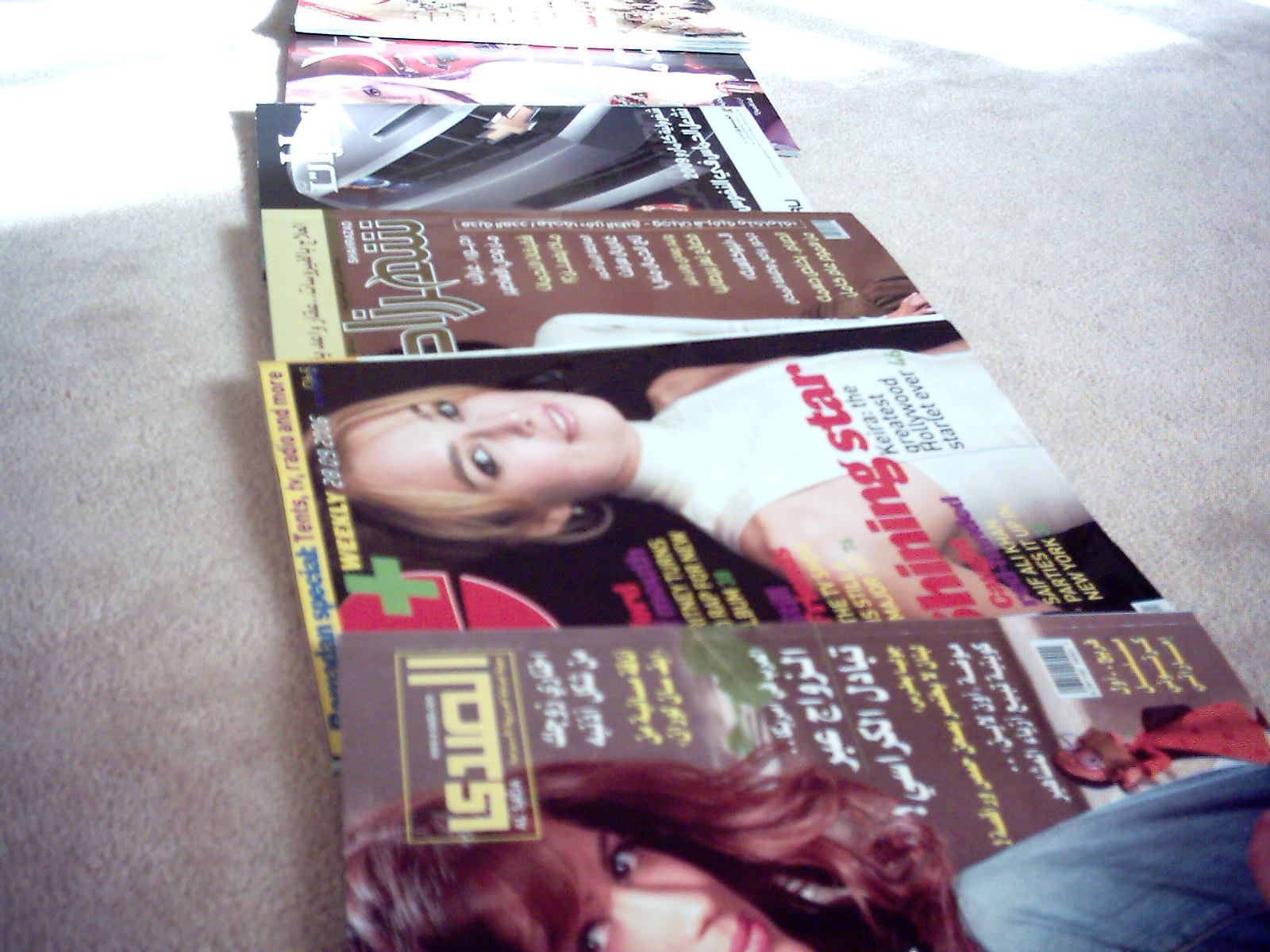A collection of seven old magazines, dating from around 2006, is carefully laid out in a single row on a tan carpet. These colorful magazines, originating from a foreign country, feature covers in either Hebrew or Arabic, though the exact language is difficult to discern. The covers showcase a variety of images and themes: two of the magazines prominently display women, one possibly featuring actress Keira Knightley, while another has a picture of a car. A particular issue set against a brown background is especially noticeable with its Arabic script. Influenced by natural light, these diverse publications hint at being part of a personal collection.